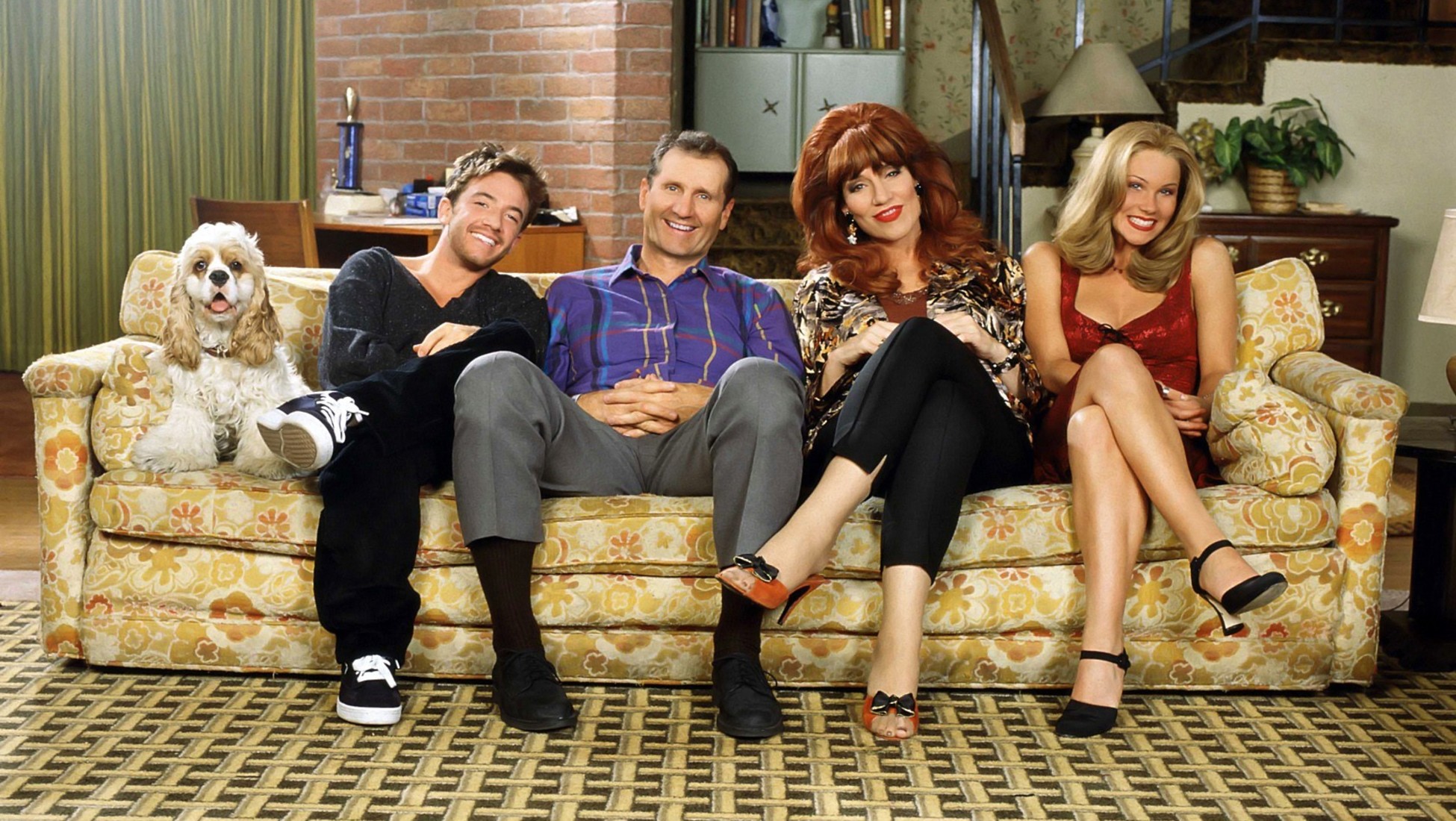This is a still photograph from the iconic sitcom "Married with Children," which was popular during the late 80s and early 90s. The image features the main cast, known as the Bundy family, seated together on a long, printed yellow and beige sofa. From left to right, the family members are positioned as follows: the dog, then the younger son who is dressed in black, followed by the father, Al Bundy, who is sporting a blue-purple striped shirt, gray pants, black socks, and shoes. Next to Al is the mother with her distinctive, voluminous red bouffant hair, wearing a printed top, black pants, and open-toed red shoes. Completing the lineup is the daughter, dressed in a revealing red top and skirt with bare legs and black pumps. The entire ensemble is staged within a typical living room set, characterized by a brick wall, green-yellow curtains, and a background featuring a staircase, a potted plant, a dresser with a lamp, and various decorative elements. The setting is complemented by an unattractive yellow and black patterned rug, accentuating the sitcom's humorous portrayal of a dysfunctional yet endearing family.